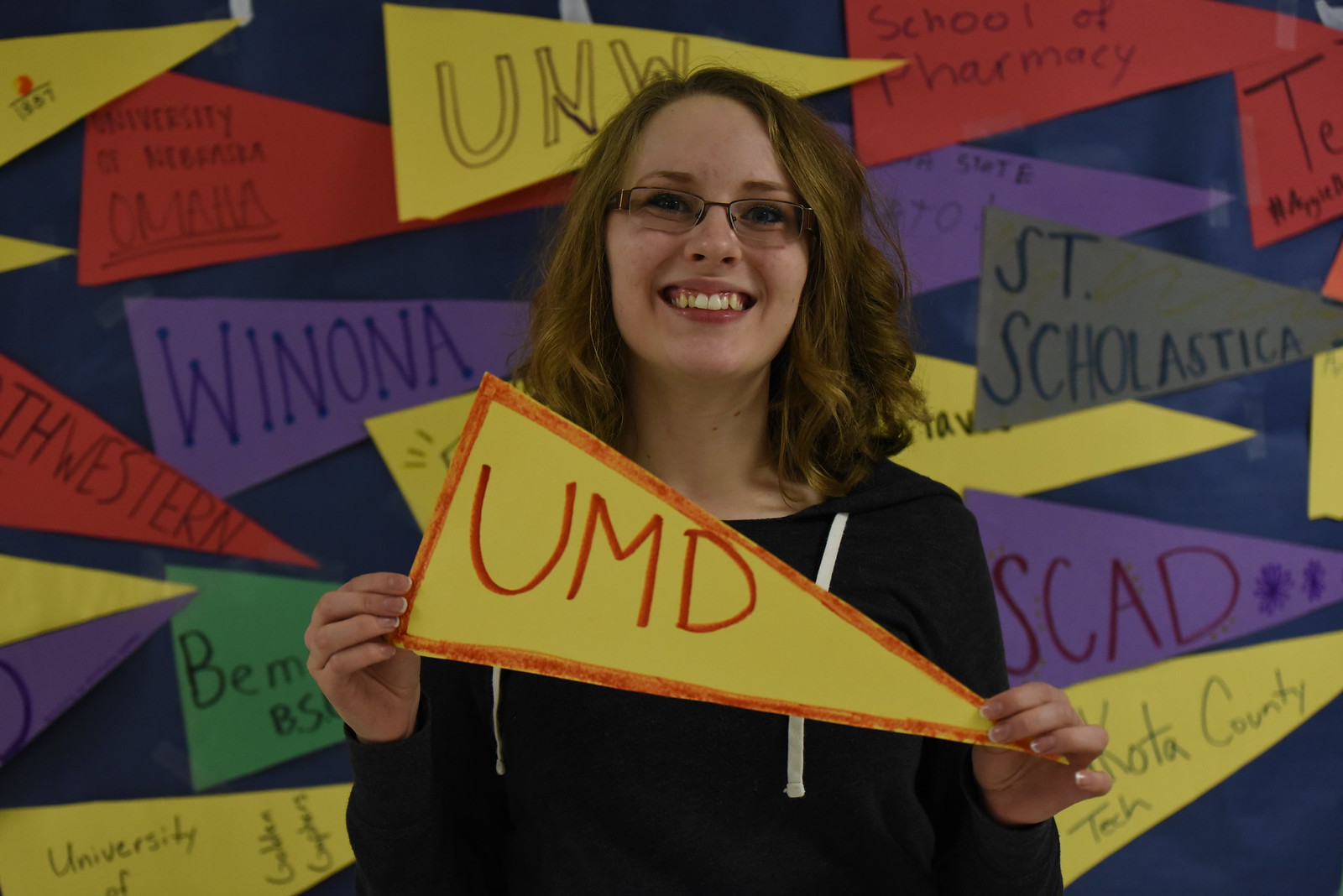This photograph showcases a smiling white woman, likely in her late 20s or early 30s, posing at the center of the image. She has curly brunette hair, wears glasses, and is dressed in a black hoodie with white drawstrings. She is holding a handmade triangular pennant cut from yellow construction paper, adorned with an orange border and the letters "UMD" written in red. The backdrop features a navy blue wall decorated with various colorful pennants, each with a different name or text. These pennants, in hues such as yellow, purple, red, and green, display names including "Winona," "SCAD," and "St. Scholastica," among others. The woman’s broad smile and the vibrant, crafted decor create a lively and cheerful atmosphere.